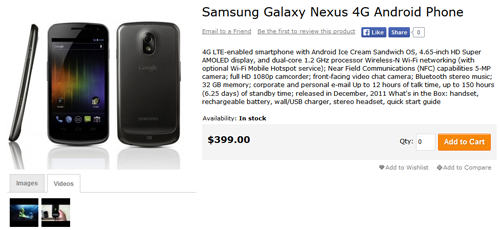This image captures a digital device displaying a listing for the Samsung Galaxy Nexus 4G Android phone. On the right side of the screen, boldly written in black font, it reads "Samsung Galaxy Nexus 4G Android phone." On the left side of the image, there is a composite image showcasing three different views of the phone. The first image provides a sideways view, highlighting the phone's thin profile. The second image, placed centrally, displays the front screen, offering a clear look at the device's user interface. The third image on the far right shows the back of the phone, detailing the camera and rear design. Below these images, there are additional thumbnail images indicating available videos. To the right of these thumbnails, descriptive text mentions key features of the device: "4G LTE enabled smartphone with Android Ice Cream Sandwich OS, 4.65-inch Super AMOLED display, and dual-core 1.2 GHz processor," followed by a continuation of technical specifications and more detailed information.